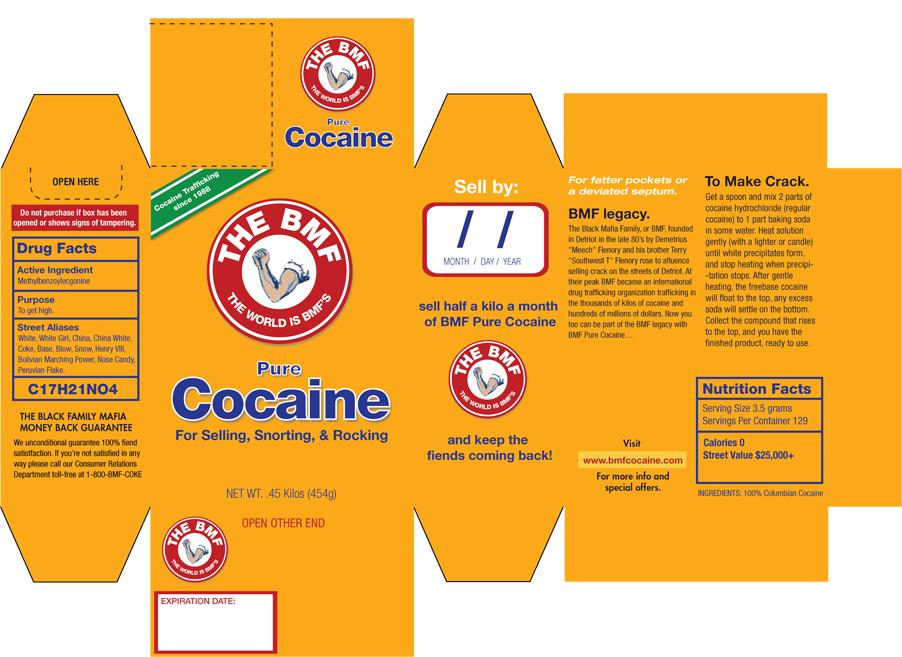The image depicts a digital illustration of an unassembled cardboard box designed to mimic an Arm & Hammer baking soda package. The background is absent, giving the impression that the image might have been cropped or taken from online. Instead of the iconic orange color, the box is a slightly more yellow hue. The front of the box features a circular red logo with a flexing arm in the center, a parody of the usual hammer, accompanied by the text "BMF" and the slogan "The world is BMF's."

The primary text on the front reads "Pure Cocaine" in large letters, with the additional phrases "For Selling, Snorting, and Rocking" underneath. There are several smaller details, including "The Black Family Mafia Guarantee" and "Nutrition Facts" in the lower right corner. The nutrition panel lists unusual data with 129 servings per container, a serving size of 3.5 grams, zero calories, and a street value of $25,000. Another section labeled "Drug Facts" mentions "Active Ingredient" and "Purpose: to get high," although much of the fine print is too small to read.

Overall, the illustration appears to be a satirical or gag gift, referencing cocaine in a humorous and exaggerated manner.